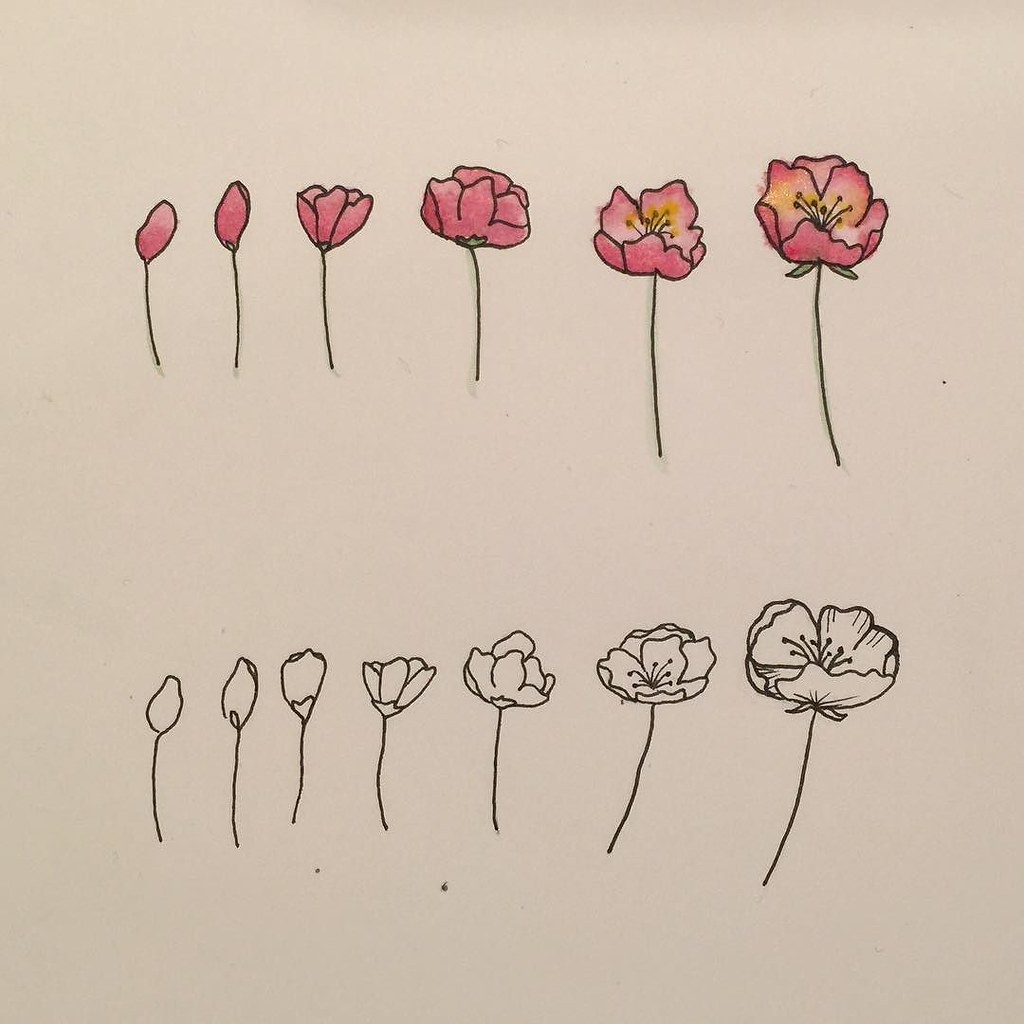The image features a delicate floral design set against a light purplish-gray background. At the bottom, a horizontal row of seven flowers is depicted, each outlined in black with the inner spaces left in the light gray color of the paper. Above them, there are six larger flowers, similarly outlined in black but filled in with shades of pink. The two flowers on the far right of this row have yellow sections within them. Each flower, regardless of row, has a distinct black vertical line serving as its stem. The arrangement and shapes of the flowers hint at botanical diversity, with tulip-shaped blooms populating the left side and rose-shaped blooms on the right.